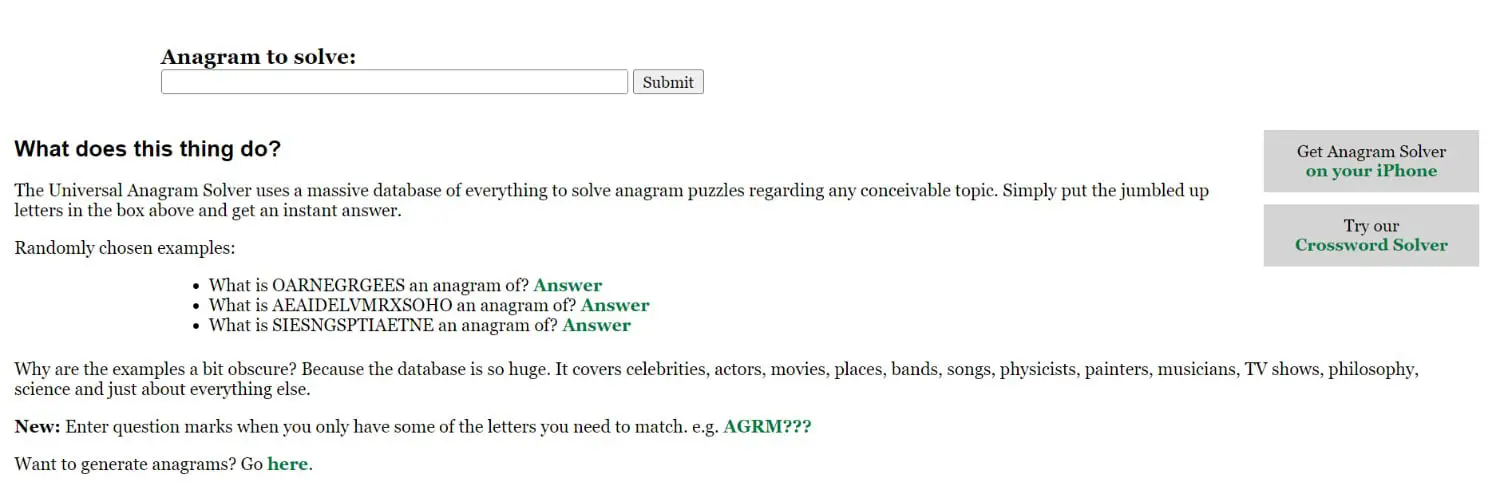This screenshot, captured from a tablet or other device, features a webpage predominantly set against a white background. Located on the left-hand side is a rectangular submission bar. Adjacent to it is a dark grey, clickable button with bold black text that reads "Submit." Above the submission bar, another line of bold black text states, "Enneagram to solve..."

On the far right-hand side of the page, two dark grey buttons are stacked. Each button displays bold black text at the top with green text beneath it. The first button reads "Enneagram solver on your iPhone" followed by "Try our crossword solver."

Further on the left, more black text asks, "What does this thing do?" It explains, "The universal algorithm solver uses a massive database of everything to solve Enneagram puzzles regarding any conceived topic. Simply put the jumbled-up letters in the box above and get an instant answer."

Below this explanation, there's another section labeled "Randomly chosen examples," featuring a list of bullet points. Each bullet point ends with an answer noted in bold green text. The examples are as follows:
- "What is the OARNEGRGESEES Enneagram of?"
- "What is AEAIDELVMRXSOHO Enneagram of?"
- "What is SISNGSPITIAETNE Enneagram of?"

A subsequent black text query reads, "Why are the examples a bit obscure?" It answers, "Because the database is so huge. It covers celebrities, actors, movies, places, bands, songs, physicists, painters, musicians, TV shows, philosophy, science, and just about everything else."

Lastly, under a "New:" section in bold black, an instructional note reads, "Enter ?'s when you only have some of the letters you need to match. E.g., AGRM???." Concluding the page, an invitation in black text asks, "Want to generate enneagrams?" followed by a clickable hyperlink in green text that says "here."

This comprehensive summary describes the layout and content of the webpage, presenting the key functions and features it offers.